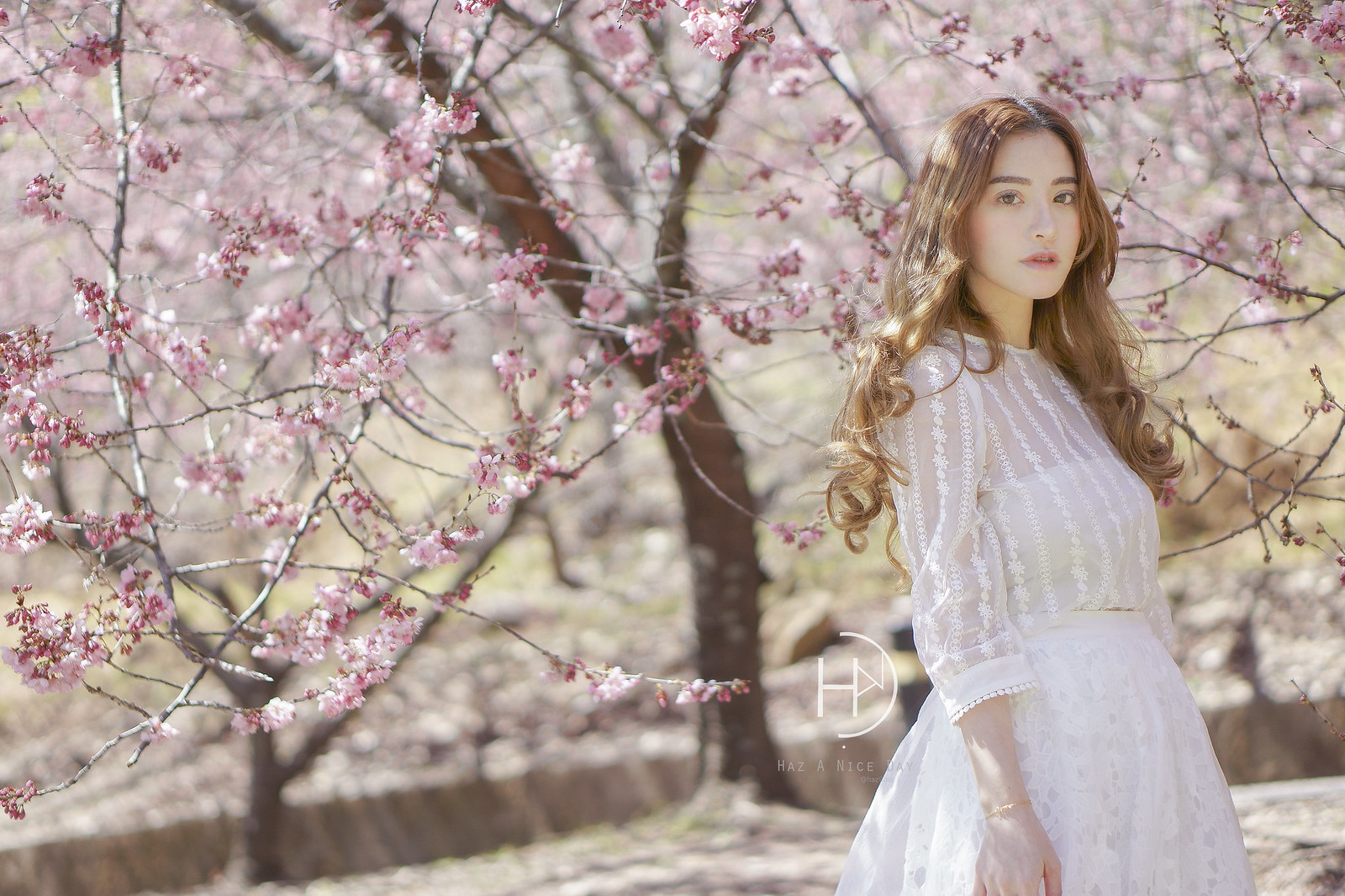A captivating outdoor photograph captures the delicate beauty of pink cherry blossoms in full bloom on three trees under a radiant sun. Dominating the right side of the image is a young girl, possibly in her early to mid-20s, with long dyed red-brown hair cascading past her shoulders. Her attire is a stunning white lace dress with sheer sleeves that delicately cover her arms and bodice, extending down to her waist. Adorned with light, natural makeup, her cheeks bear a subtle rosy hue that complements her pink lips. She wears a delicate gold bracelet on her wrist. Her expression is a mix of forlorn surprise, directing her gaze either at the camera or something unseen in the distance. To the left of this striking figure, an emblem features the letters "H," "A," and "V" within a semicircle, accompanied by the phrase "Have a nice day." The ensemble of the enchanting cherry blossoms and her poised presence creates a serene yet evocative scene that hints at a deeper narrative.